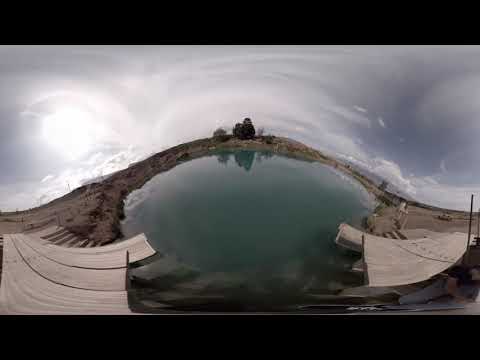In the image, at the center, there is a small, aqua-colored lake surrounded by a combination of sand, dirt, and grassy areas, creating a natural, serene landscape. Towards the bottom, a wooden dock extends into the lake, complete with stair steps on its left side. Scattered pieces of long wood can be seen on the sandy ground to the left of the water. Framing the scene, there are a few trees around the perimeter and in the background, along with a small brown building atop a hill. The sky is largely overcast with numerous clouds, giving the impression of an impending rain shower. The sun is low on the left side, casting a partial halo likely due to precipitation or a potential rainbow. In the distance, mountains rise on the center right, contributing to the picturesque outdoor setting captured in what appears to be the middle of the day. No people are present, and the scene is devoid of text, emphasizing the tranquil, natural beauty of the location. The color palette includes shades of black, gray, white, green, tan, blue, and aqua, enriching the detailed composition of the image.